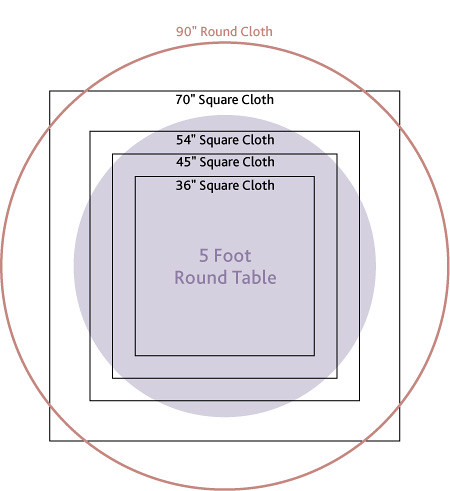The image displays a series of concentric squares and circles, each labeled with specific measurements and descriptions. 

1. At the center, there is a square labeled "36 inch square cloth."
2. Surrounding this is a larger square labeled "45 inch square cloth."
3. The next layer is an even larger square marked "54 inch square cloth."
4. Further out, there is a gray circle containing the text "5 foot round table."
5. Beyond this, there is another square labeled "70 inch square cloth."
6. The outermost shape is an orange circle labeled "90 inch round cloth."

Each layer visually represents a different size of cloth or table, providing a clear comparison of their dimensions.